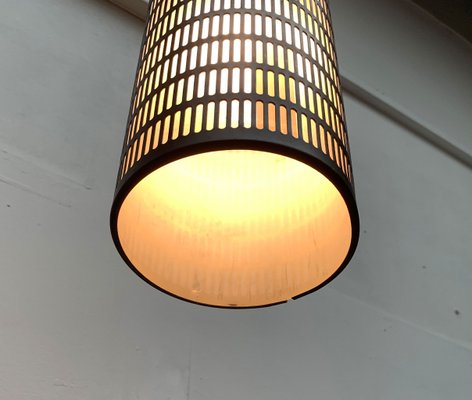The image captures a very close-up photograph of a cylindrical light fixture with a black metal finish. The light is turned on, casting a vibrant, glowing amber and yellow light. This cylindrical fixture features a pattern of small, oval-shaped perforations encircling its surface, allowing light to seep through, and it culminates in a large circular opening at its base, highlighted by a thick black trim. The background is a smooth white concrete wall, although it's not clear whether this fixture is a wall sconce or a pendant light. The overall environment is dim, emphasizing the vivid illumination from the light, whose interior glow transitions subtly from yellow to orange. The detailed texture and color gradients inside the lamp add to its captivating appearance, despite its attachment point being out of view.